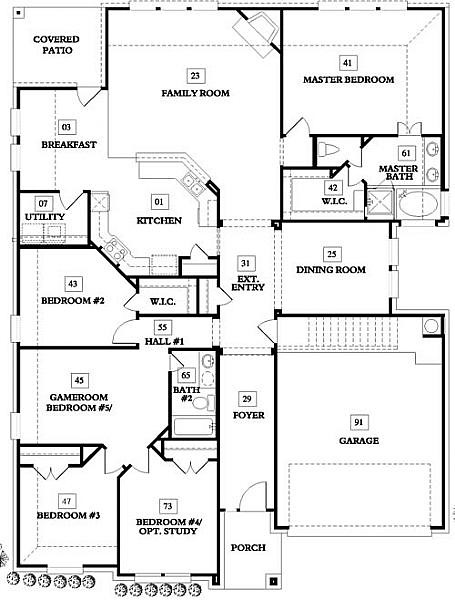This detailed architectural blueprint illustrates the layout of a spacious, one-level house. At the top of the blueprint, the house features a covered patio, a large family room, and the master bedroom. Directly beneath the master bedroom is the master bathroom, complete with a walk-in closet. Below the family room, centrally located, are the kitchen, entryway, another walk-in closet, and a hallway. Adjacent to the covered patio on the right, the blueprint shows a breakfast nook, kitchen, utility room or utility closet, and an additional bedroom.

In the bottom half of the blueprint, the right side prominently features a large garage, which occupies more space than the family room. Next to the garage, there's a foyer and a porch. Further to the left of this area is the second bathroom, bedroom number four which can also serve as an optional study, and nearby, bedroom number three. Additionally, there is a versatile space that can be used as a game room or another bedroom, offering flexible living arrangements. This comprehensive blueprint provides a clear, top-down view of the home's thoughtful and functional design.